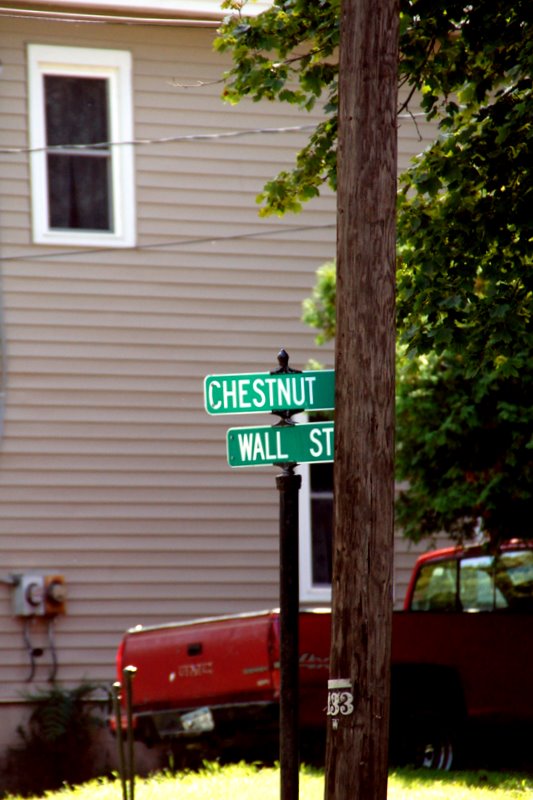This outdoor photograph captures a street sign mounted on a black metal pole, approximately eight feet tall. The sign includes two horizontally oriented rectangular panels. The panel facing the camera is green and white and prominently displays "Wall Street." Adjacent to it, partially obscured by a large brown utility pole, is another sign that likely reads "Chestnut Street," although only "Chestnut" is visible. In the background, there is an older model red GMC pickup truck, suggesting the photo may have been taken some years ago. Further back, a house with white horizontal siding and several bushes in front can be seen, providing a suburban context to the scene.